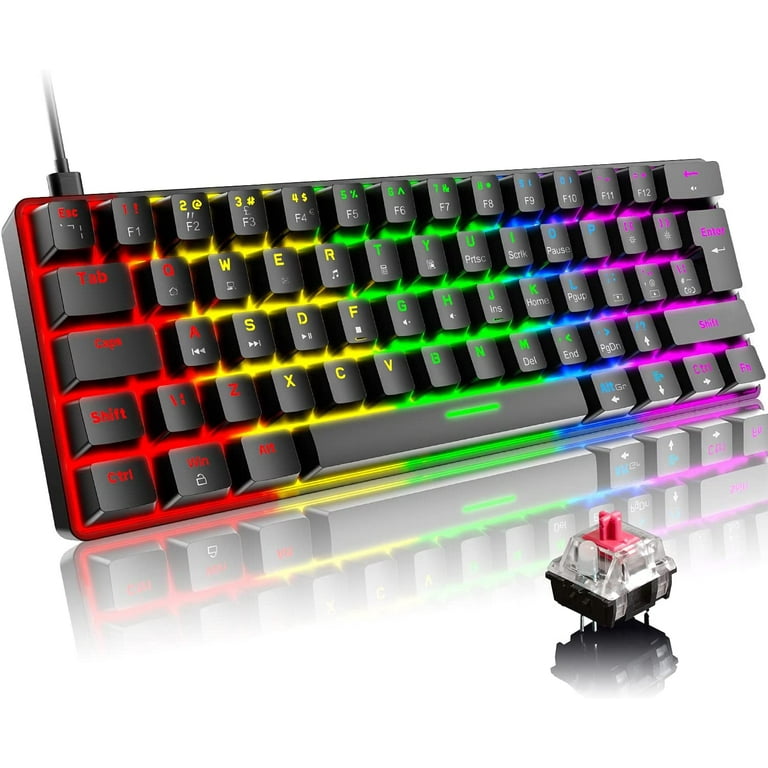This photograph features a visually striking, fully backlit keyboard standing upright on its bottom edge. The keyboard is illuminated with a vibrant, rainbow gradient of colors that transition from red on the left, through yellow, green, blue, and finally to purple on the right. Each section of keys matches the background color, with the keys themselves being black and the letters lighting up in the corresponding colors. For example, the keys on the left, including 'Caps Lock', 'Shift', and 'Tab', are illuminated in red, while keys on the opposite end, such as 'Enter', 'Shift', and 'Control', are bathed in purple light. 

To the upper left of the image, a cable is visibly connected to the keyboard, and the surface below reflects the colorful light, creating a mesmerizing mirrored effect. In the bottom right of the photograph, there is a small, clear, black, and red plug or electrical object also reflected on the surface. The foreground prominently features a detailed view of the inner mechanism of a keyboard key—showing the connectors, spring part, and an LED light—indicating this may be an advertisement for customizable backlit keys.